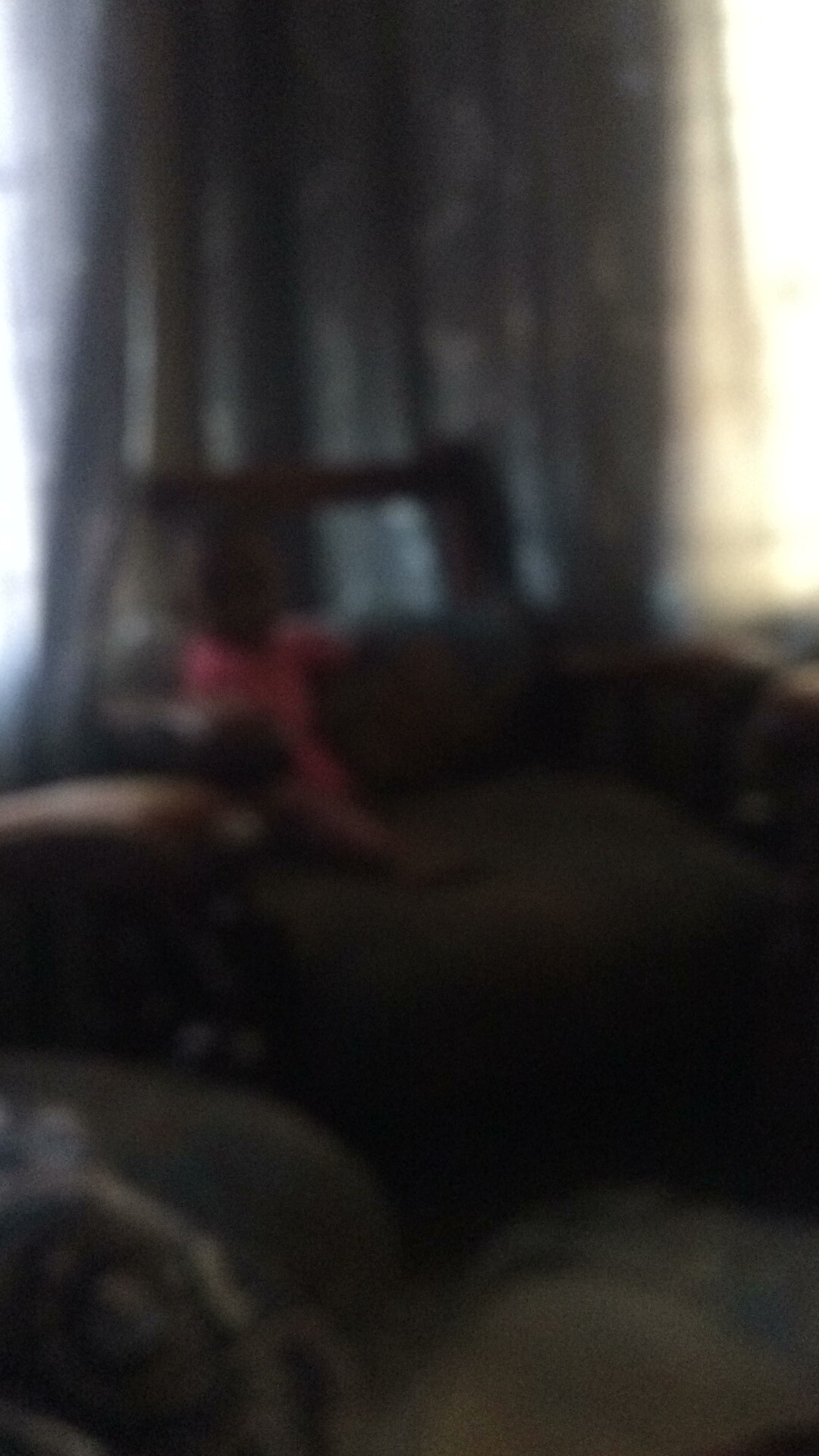This image is a very blurry and out-of-focus photo of an indoor setting, likely the living room of someone's home. Dominating the background are large, dark gray curtains that obscure the windows, casting the room in a dim light. Some light manages to seep through, creating a faint yellowish hue along the edges of the curtains. 

In the center of the image, there appears to be a dark gray couch or recliner with a prominent, cushy seat and a low backrest. Seated on this piece of furniture is a small child, possibly African-American, who is dressed in a pink top and pink shorts. Although the overall image is indistinct, there's a noticeable depiction of the child’s legs dangling from the seat. The room's overall dimness and the persistent blurriness make it challenging to discern finer details.